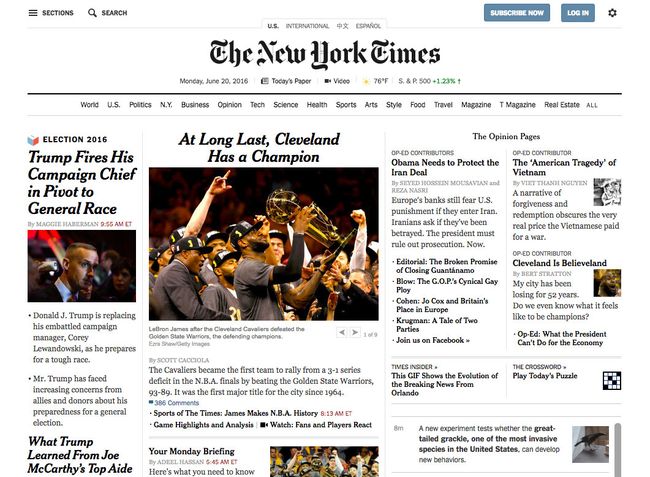The image captures the homepage of the New York Times website. In the top left corner, there is a black icon with three horizontal bars labeled "Sections," adjacent to a magnifying glass icon labeled "Search," both in black text. On the far right, there are two blue boxes with white text; one reads "Subscribe Now" and the other "Log In." Dominating the top center of the screen is the prominent New York Times logo. The homepage features multiple headlines and brief synopses. On the left side of the image, an article headline reads "Trump Fires His Campaign Chief in Pivot to General Race," under the Election 2016 section, indicating the content’s older date. In the center, another headline declares "At Long Last, Cleveland has a Champion," accompanied by a photo of LeBron James proudly holding a large trophy.